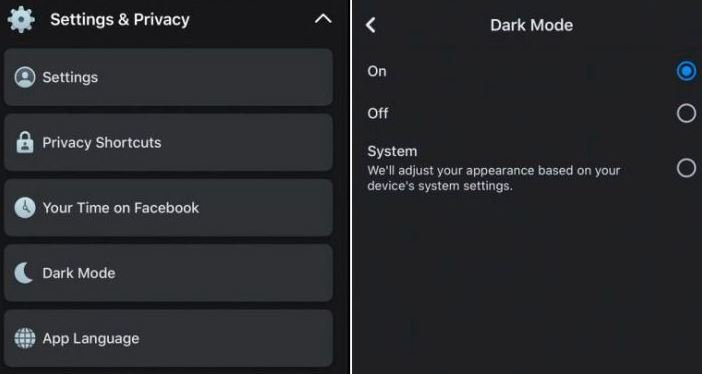In the image, a user is navigating through their settings on a mobile app. The interface is configured with dark mode enabled, featuring a sleek black background and contrasting white text for readability. The settings panel showcases several options including "Privacy Shortcuts," "Your Time on Facebook," "Dark Mode," and "App Language," among others. The overall aesthetic is minimalist and clean, allowing for easy navigation and user customization.